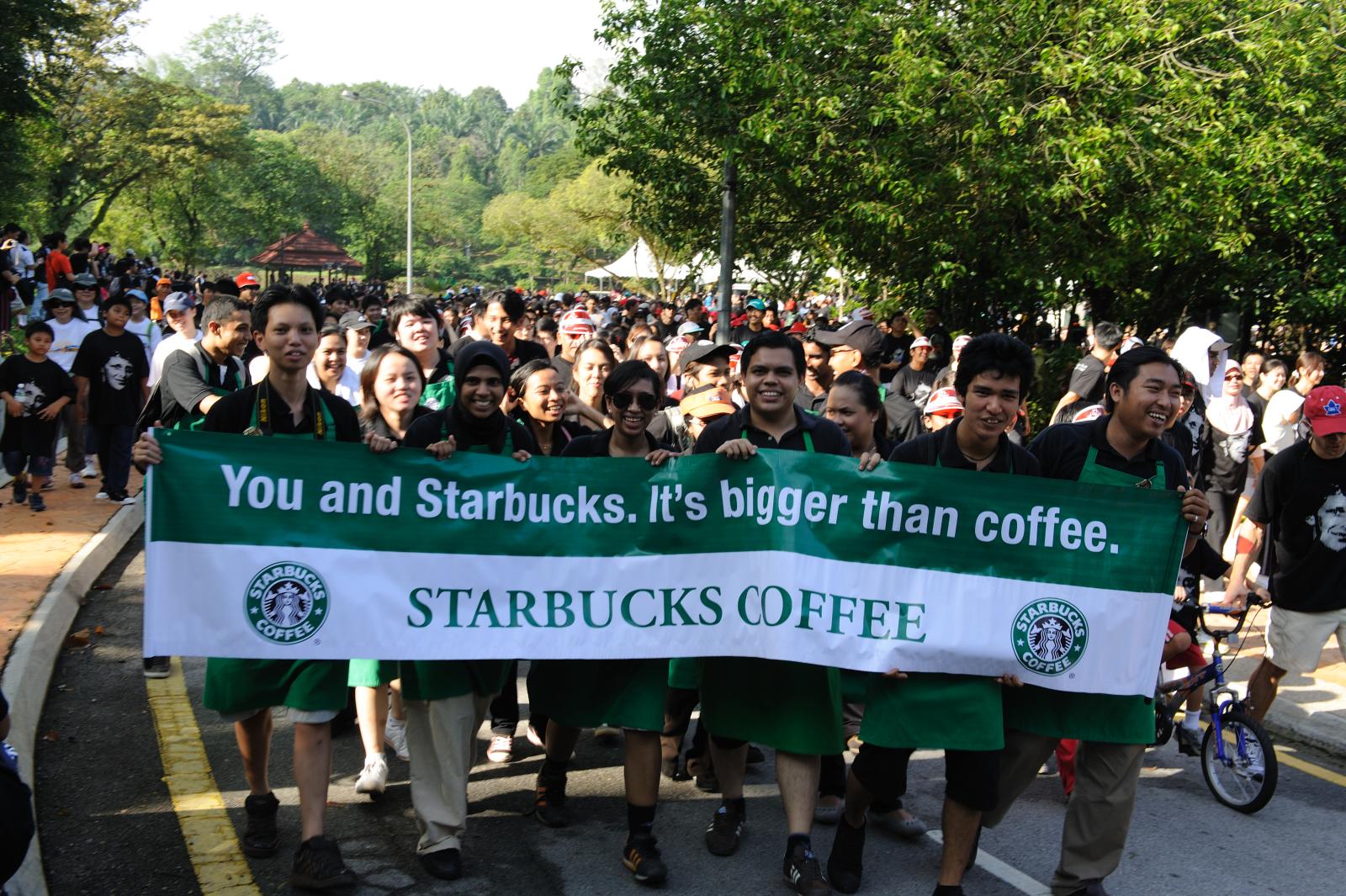In this vibrant photo, a group of six enthusiastic youths lead a parade, each beaming at the camera as they hold a prominent green and white banner. The upper portion of the banner, designed with white text on a green background, reads, "You and Starbucks — It's bigger than coffee." Below, the text transitions to green letters on a white background with the iconic Starbucks logo flanking the words "Starbucks Coffee." 

The parade stretches out behind them, with a diverse crowd filling the frame, including a small child on a tricycle being guided by an adult to the right. This lively scene unfolds on a bright, sunny day, evident from the vivid greenery of the surrounding trees and the crisp clarity of the street markings. In the distant background, numerous participants march onward, set against a picturesque backdrop of white tents, lush forest, and possibly a building on the left side. This gathering, potentially taking place in an Asian country, showcases a community coming together in a shared activity, unified under the banner of Starbucks.